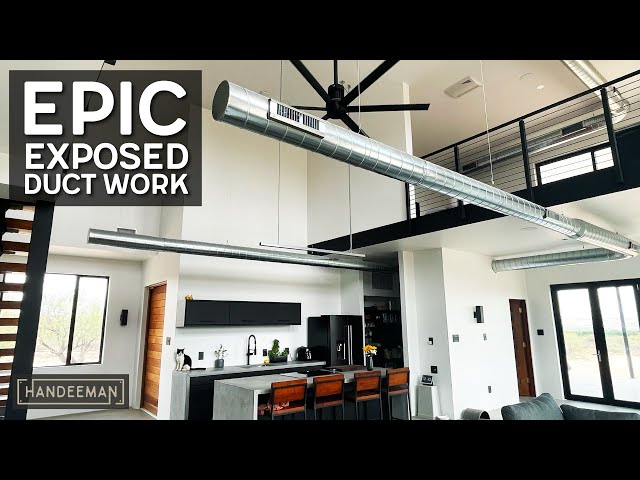This horizontal image captures a modern, open-concept kitchen extending into a living room, characterized by its tall white walls and expansive layout. Central to the design is a large black ceiling fan and prominent exposed silver ductwork that runs above the kitchen. The kitchen features a central counter with four brown chairs, a large sink, a refrigerator, and black cabinets. A balcony overlooks the ground floor, giving a clear view up to the second story, emphasizing the room’s lofty ceiling. To the upper left, the image displays overlaid white text in a gray box stating "EPIC Exposed Ductwork," with "HANDYMAN" marked in the bottom left corner. Additionally, a small section of a couch is visible in the bottom right corner, adding to the homey atmosphere of this modern design.